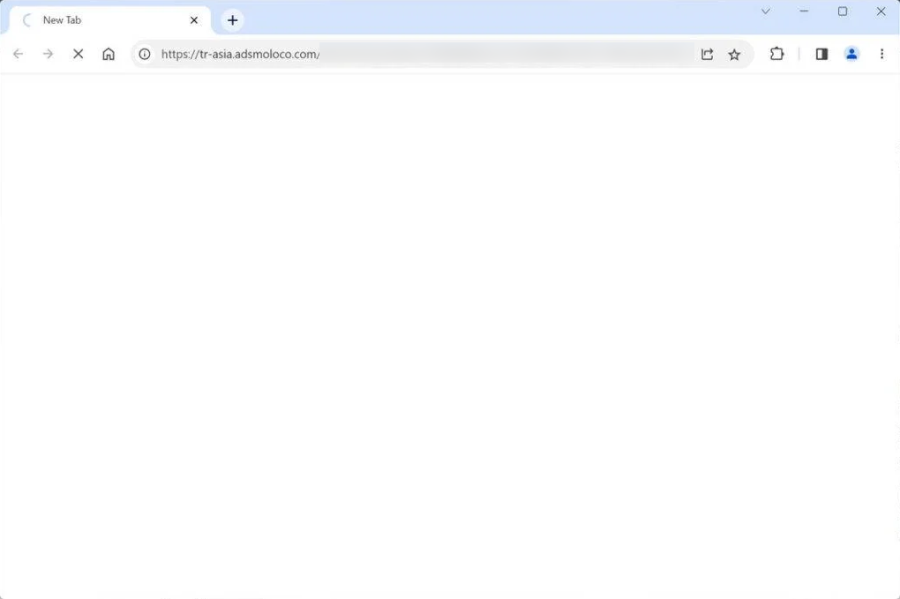This screenshot captures a webpage that has failed to load correctly. Dominating the screen is a blank browser window with a "New Tab" label at the top left. Indicating an ongoing loading process, a grey circle rotates incessantly beside the label. The address bar at the top reveals the intended destination: https://trasia.adsmoloco.com, a URL suggestive of an advertising-related platform. The rest of the screen remains starkly empty, with no page content displayed. Standard browser window controls, including minimize, fullscreen, and close buttons, are visible in the top right corner.